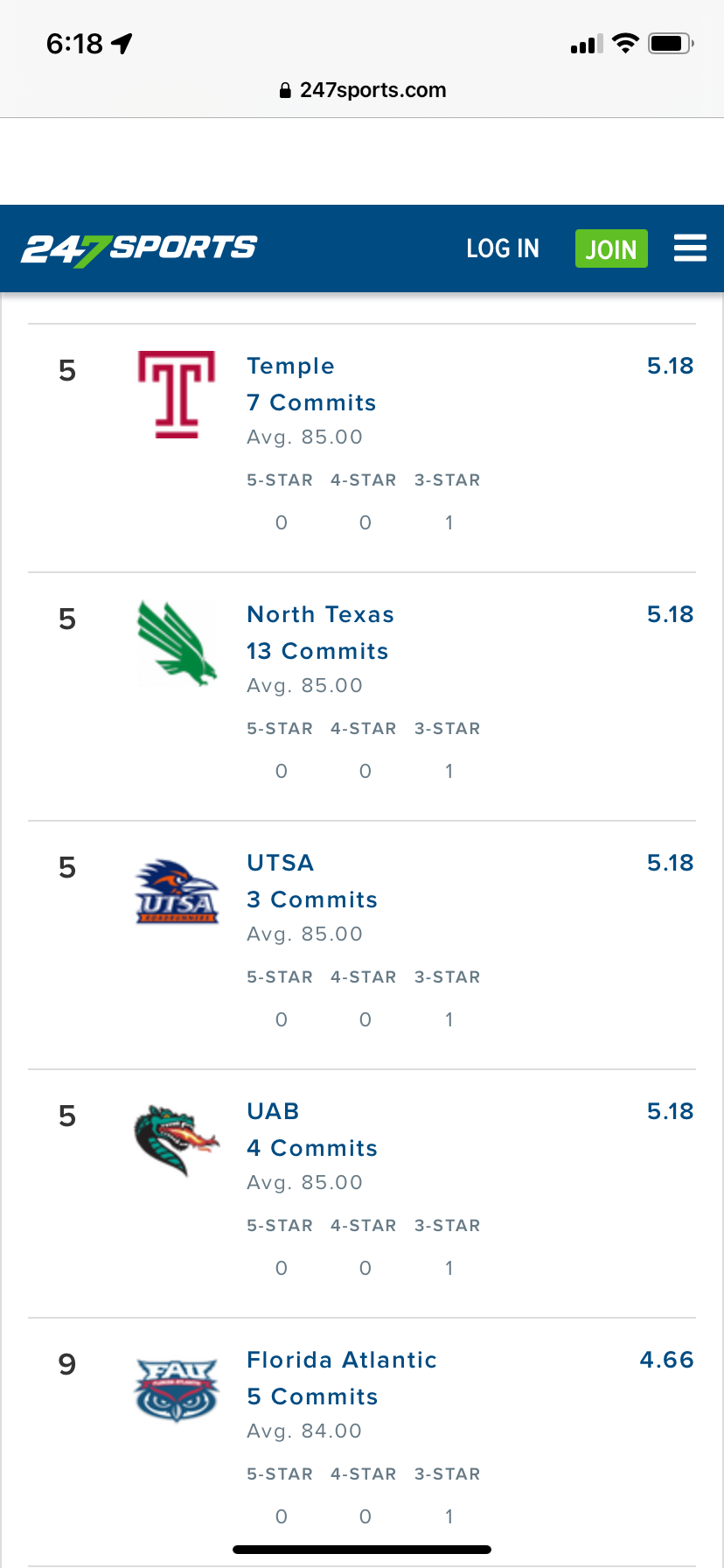A detailed screenshot image shows the top section of a smartphone screen, taken at 6:18 PM. The status bar displays various indicators: a location tag resembling an airplane at a 45-degree angle, three out of four bars of cellular service, full Wi-Fi signal, and a nearly full battery estimated to be between 85-90%, with a solid black battery icon but no percentage displayed. A small lock icon is also present. 

Beneath the status bar, there is a URL in black font on a light gray background, reading "24-7sports.com". Below a subtle divider, a navy blue rectangle features the "24-7 sports" logo with '24' and 'sports' in white font, the numeral '7' in lime green. Adjacent to this, in white font, 'login' is visible. A smaller green rectangle with 'join' in white font and three parallel lines appear alongside the main logo.

The main section exhibits a series of sports team logos and relevant information, highlighted by icons and names: Temple, North Texas, USTA, UAB, and Florida Atlantic, accompanied by repeated values of '5, 5, 5, 5, and 9', likely representing team statistics or rankings. This collection of elements provides a comprehensive snapshot of a sports-related webpage displayed on a smartphone.